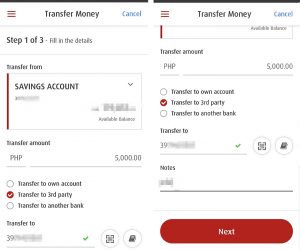In this image, the user interface displays the first step of a three-step process for transferring money. The form prompts the user to fill in details for the transfer. Specifically, it shows options to transfer from a savings account, with an amount of $5000 indicated. The transfer is set to be made to third-party accounts, specifically to another bank. Certain sensitive information, like the receiver's or sender's personal details, is intentionally blurred to protect privacy. The overall design features a red, blue, and black color scheme against a clean white background.